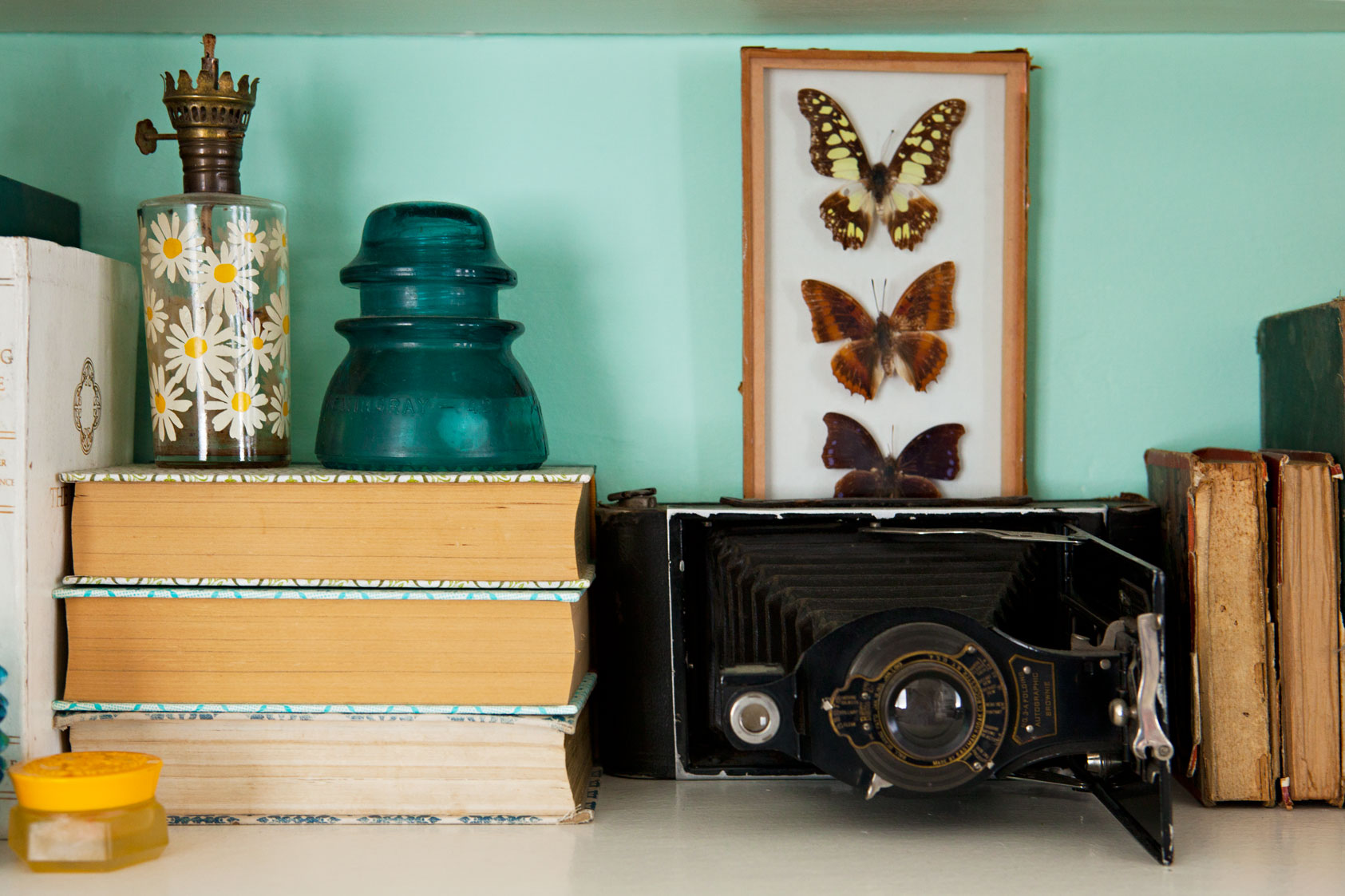In the photograph, a light gray, shiny countertop reflects a neatly arranged collection of items against a pale mint-colored wall with a light gray stripe at the top. Starting from the left, a series of books capture attention: a white book peeks out from the left edge, partially obscured by another book. Adjacent to these, three books lie flat, displaying their brownish pages with the bindings pressed against the wall. In front of these books, a small, semi-transparent jar with a yellow top is visible.

On top of the stacked books, there's a cylindrical jar adorned with white flowers and yellow centers, capped with a copper-finished lid resembling a crown, featuring a small knob on the left side. Beside it, a teal glass object adds a touch of color. Moving towards the right, an old-fashioned black camera, characterized by its accordion-like bellows, sits prominently on the countertop. It features an extending lens with an additional smaller encased lens on the left.

To the right of the camera, two well-worn, brown books stand upright with their yellowing pages exposed vertically. Behind the camera, a wooden-framed picture showcases three brown butterflies against a white background, with the bottom butterfly partially hidden by the camera. The overall composition of books, jars, and the antique camera, set against the cool-toned wall, creates a nostalgic and visually harmonious arrangement.